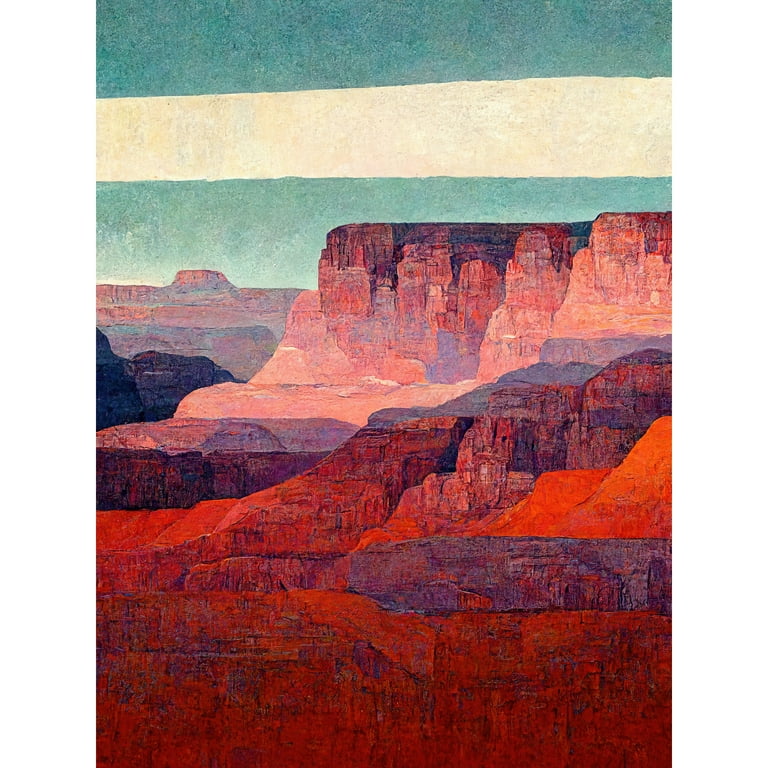The painting is a detailed, rectangular-shaped landscape illustration of what resembles the Grand Canyon's rocky desert terrain. It features striking, layered mountains with distinct, flat tops and varying colors, predominantly shades of red, brown, and peach. The lower section of the mountains is intensely red, transitioning upwards through dark red to light and dark brown hues. The rocky formations exhibit a jagged, rugged texture, with sheer drops and taller peaks towards the center. The sky above is characterized by a teal hue, interrupted by a beige horizontal stripe, adding to the picturesque and somewhat surreal quality of the scene. The painting exudes a textured look, enhancing the vibrant, dry, and vegetation-free canyon landscape.